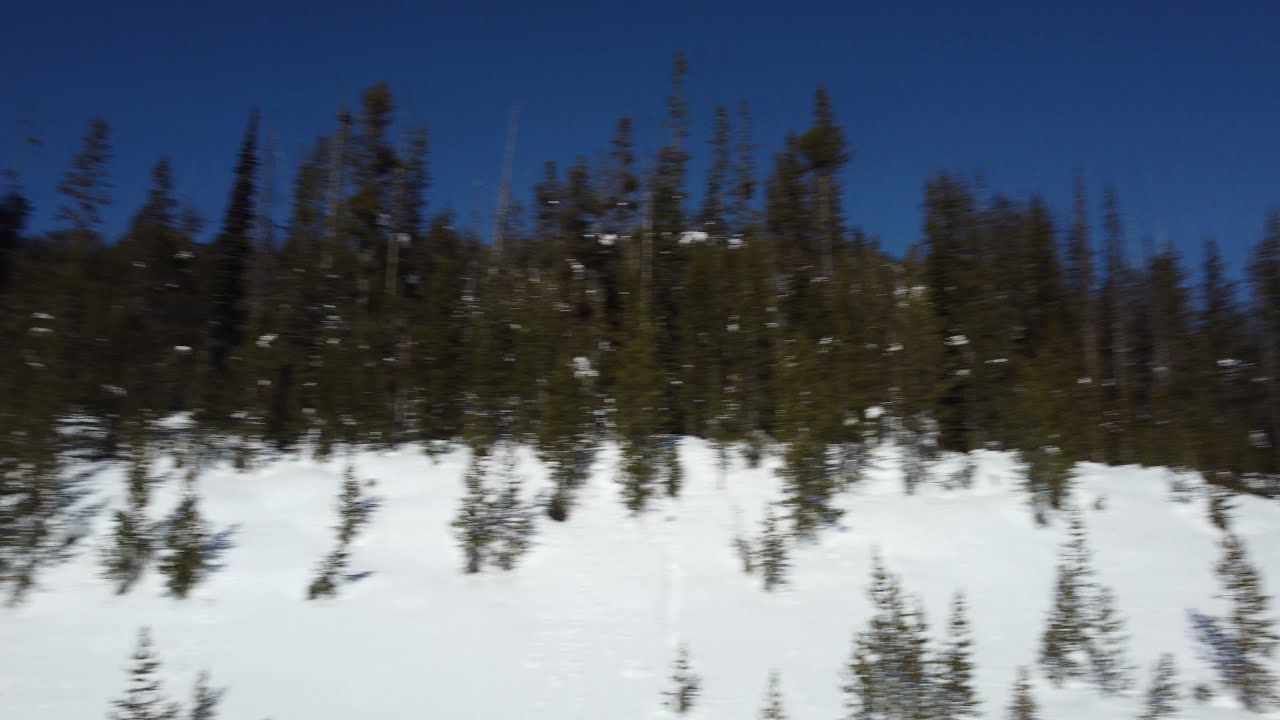This photograph captures a serene, snowy hillside landscape viewed from below. The composition is divided into three horizontal sections. The bottom third features a snowy blanket with scattered short pine trees, their presence faintly outlined in the snow. Moving upward, the middle third reveals a dense forest of tall and short pine trees, their green needles lightly dusted with snow. The top third is dominated by a dark navy blue sky, suggesting dusk or early evening. The image exudes a calm, wintry atmosphere, with the dark forest backdrop adding depth and a sense of stillness to the scene.